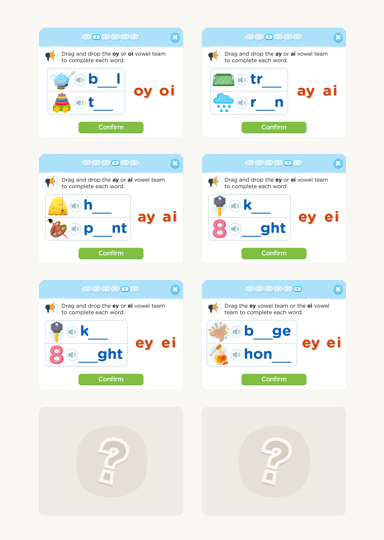This is a detailed screenshot of a children's language-learning app. The interface is structured into two columns, each containing four boxes. The boxes follow a consistent design, featuring a light blue header with navigation buttons at the top, and a white body. 

In the first box, a speaker icon and the instruction "Drag and drop the O-Y or O-I vowel below to complete each word" are displayed. Below this instruction are images of a teapot and a stacking toy. Next to each image, there are speaker icons and partially completed words: "B__L" for the teapot and "T__Y" for the toy. The child is given two vowel choices, "O-Y" and "O-I," both highlighted in orange. A green confirm button is located at the bottom of the box.

The same format applies to the other boxes, except the last two, which are marked with question marks and are blank. For example, the box in the second column, third row, instructs the user to "Drag the E-Y or E-L vowel and complete each word." The accompanying images are a beige color and honey. The vowel choices "E-I" are highlighted in orange, and there is a green confirm button at the end.